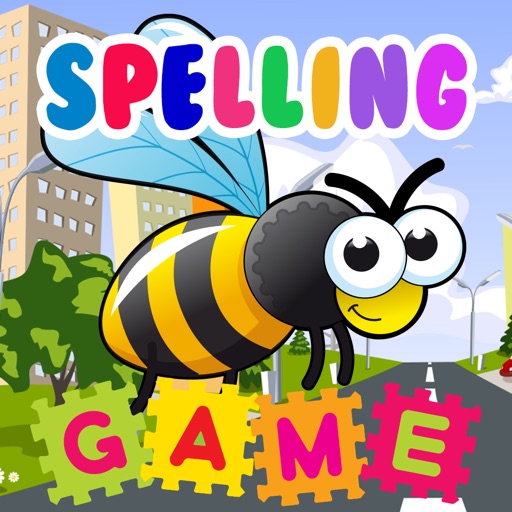The image is a colorful and engaging thumbnail for a free-to-play app game titled "Spelling Game" available on the Google App Store. The top and bottom of the image feature the words "Spelling Game," with each letter in vibrant colors like red, blue, pink, green, yellow, purple, and orange, reminiscent of bubble lettering. At the center of the image, a cheerful, cartoonish bee with big white eyes and a half-smile is flying. The bee, which has yellow and black stripes and bluish wings, is depicted in a whimsical and childlike manner. The background showcases a lively cityscape with a gray street marked by white lines, tall street lamps, green trees, and expansive green grass. Two tall brown buildings rise prominently in the background, with added details like clouds enhancing the playful, animated environment. This eye-catching, educational game thumbnail is designed to capture and hold the attention of young children.